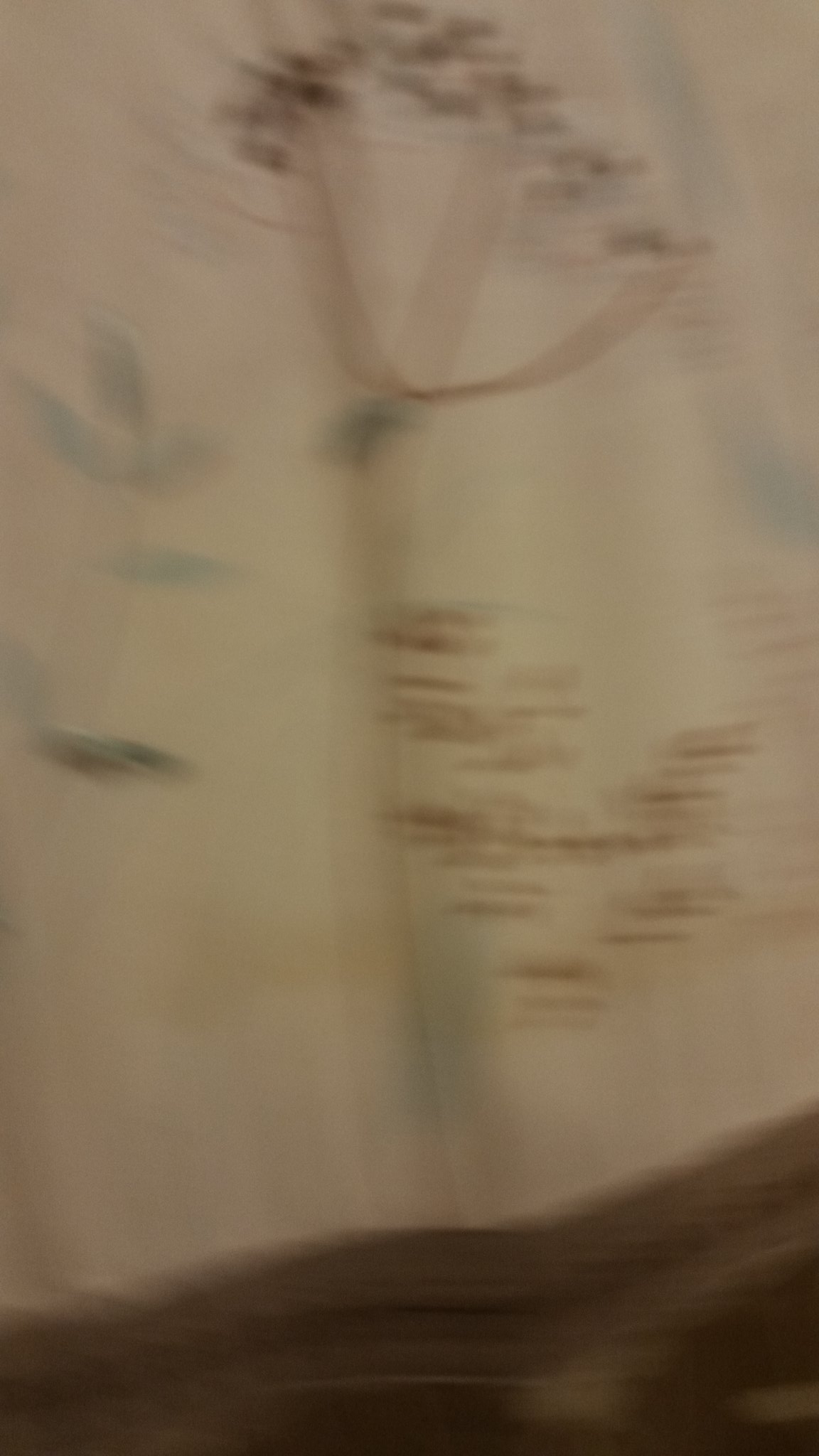This rectangular color photograph, though quite blurred and of low resolution, depicts what appears to be a children's drawing or a pattern resembling a tree on a beige background. The lighting is artificial and low, making the image difficult to discern. About 80% of the image from the top down consists of a beige area featuring brown branches with smaller brown leaves at the top. The middle and lower parts of the image include various small, brown horizontal lines, contributing to a somewhat messy appearance. To the left, there seems to be a greyish-green leaf pattern, possibly resembling birds or another plant. The bottom section of the image shows a brownish-grey, wavy triangle shape extending from the bottom left corner, curving slightly due to crumpling of the material above. Despite the blur, it suggests a scene rendered in soft colors—browns, greens, and possibly subtle blues—on a light tan backdrop, evoking an abstract, almost dreamy feel.